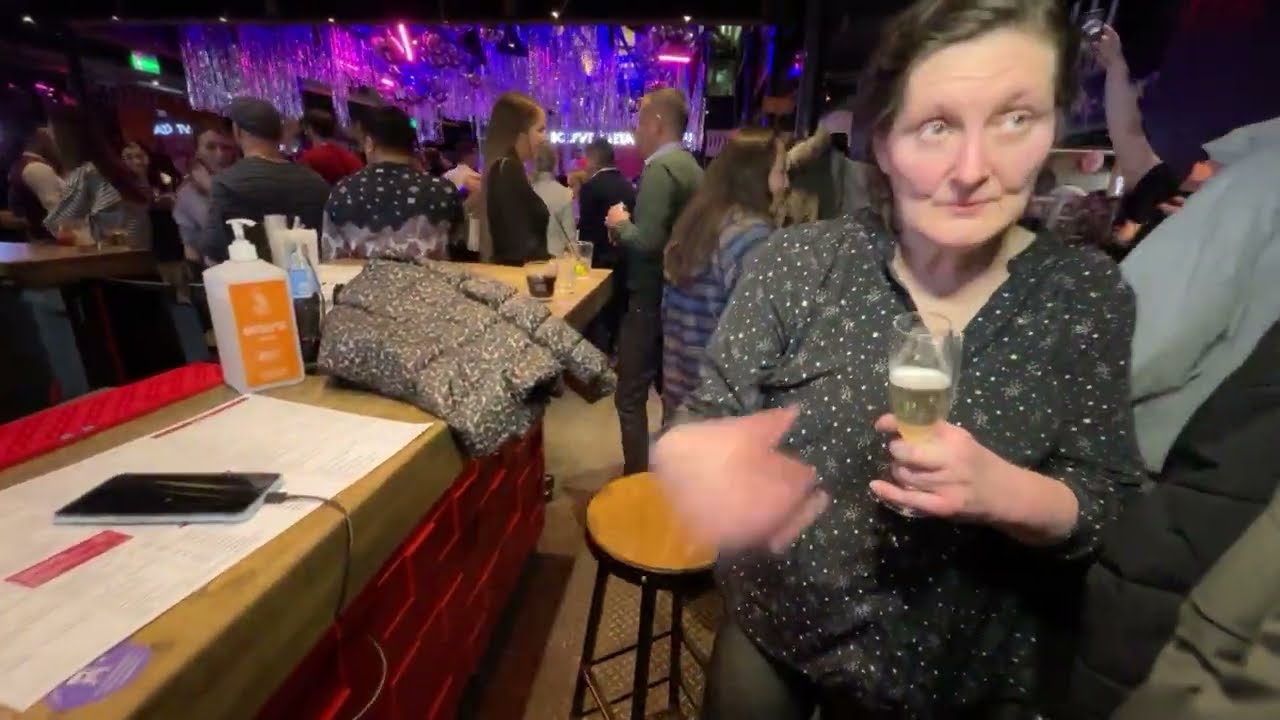In this photo, likely taken at an office party or a bar event, a light-skinned woman stands prominently in the foreground on the right holding a glass of champagne. Her champagne glass is fluted and filled with a light, golden-hued liquid. She is dressed in a gray shirt adorned with multi-colored dots, paired with dark pants. Her facial expression is neutral, and she gazes off to the right of the photograph. Her brown hair frames her face.

To the left of her, there is a bar area with a light wood finish on top and a red brick-like base. An iPad sits charging on a stack of papers atop the bar, beside a gray jacket. There's a beige-topped bar stool nearby, adding to the casual atmosphere. Drinks and large containers, possibly for hand cleaner, are also visible.

In the background, the photo captures a lively crowd, with people standing around and talking, some holding cups. The scene is dimly lit, especially towards the left side, creating a cozy ambiance. A stage, adorned with silver streamers and illuminated with purple lights, is visible in the distance, suggesting a festive environment. A yellow or greenish rectangular area is also noticeable on the left side of the image. The dark, slightly out-of-focus surroundings add depth, making the central figures stand out.